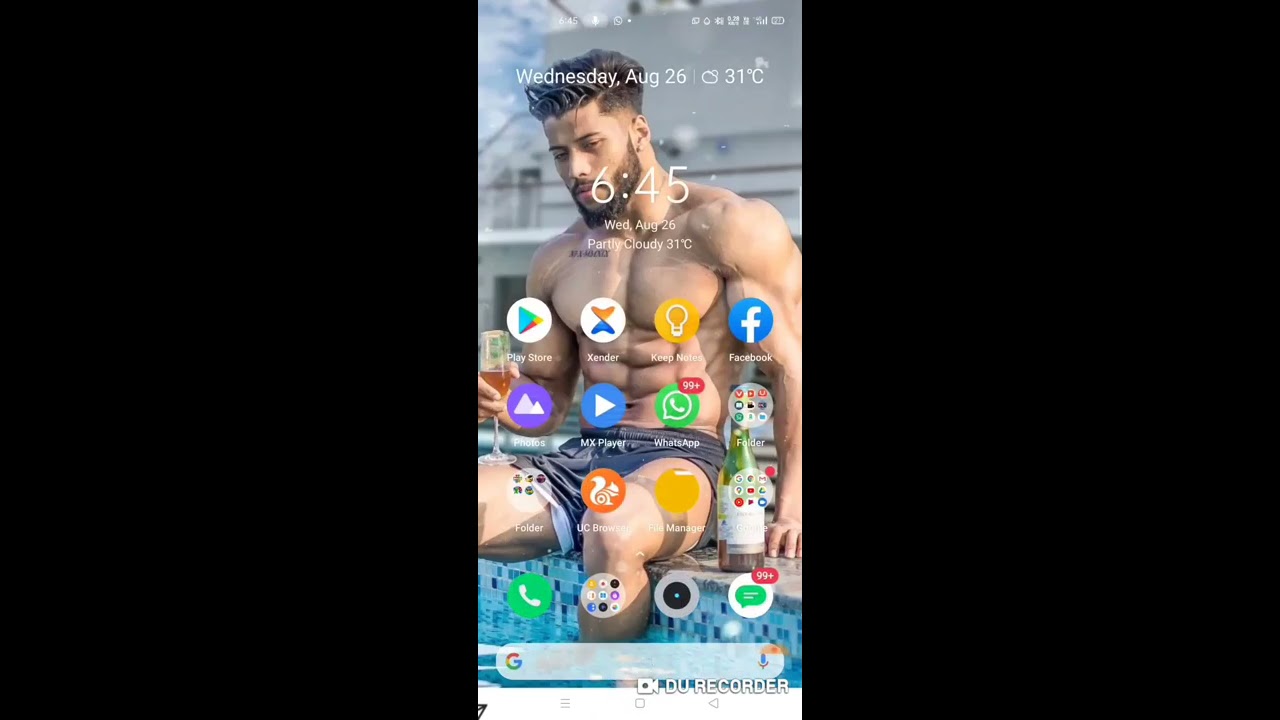The image displays a screenshot of a phone’s home page with a background featuring a shirtless, muscular man with a brown beard and wavy hair, longer on top and shorter on the sides. He is sitting on the edge of a blue pool, dipping his legs in the water, and wearing blue shorts. The man is holding a glass of an orange-ish liquid, likely champagne or wine, in his right hand, while a bottle of the same drink is placed on his left side. At the top of the screen, the date is shown as Wednesday, August 26th, and it indicates a weather condition of partly cloudy with a temperature of 31 degrees Celsius. Iconic phone features are visible, including the battery level, time stamp of 6:45, and various app icons such as the Google Play Store, Facebook, Zender, Keep Notes, Photos, MX Player, Whatsapp, and DU Recorder. The phone appears to be either a Samsung or another Android device, identifiable by the layout and presence of specific app icons. The screen is framed by wide black borders on the left and right sides.